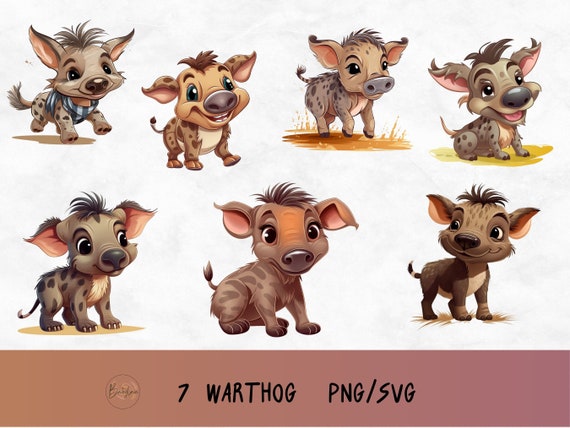The image is a detailed cartoon illustration featuring seven adorable warthogs in different poses spread across a landscape format. At the bottom section of the drawing, there's a logo that appears to be in script and reads "BRIDGES," followed by the black text "7 warthog PNG/SVG," indicating it can be used as a graphic or cut file. 

The warthogs, which resemble a mix of pigs and ponies, are depicted in hues of brown and tan, with variations in darkness; notably, the warthog on the bottom left is much darker than the others. Each warthog has big, bright eyes and tufts of hair on their heads. Their wide ears generally extend outward from the head, except for the top-left warthog, where the ears move upward diagonally like a dog's. They all feature spots of varying shades and have distinctively adorable looks, some smiling with visible teeth. 

In the top section, the warthogs are depicted running, skipping, walking in grass, and sitting. Meanwhile, in the center and bottom sections, they are illustrated standing, sitting, and looking left.